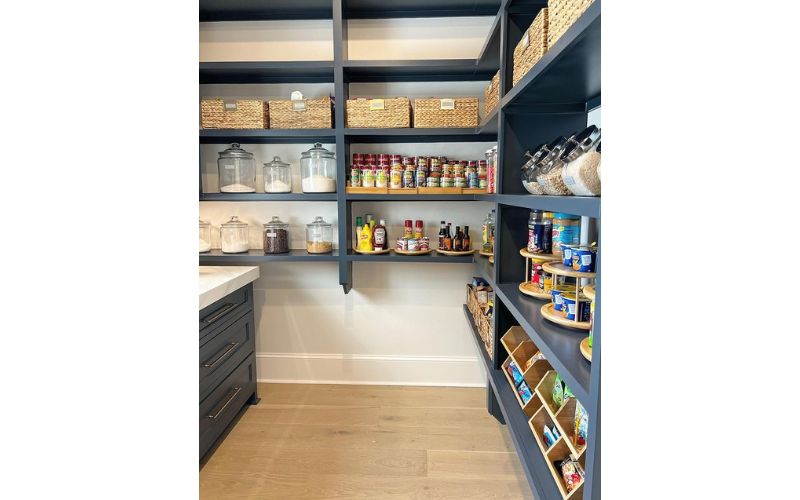The image captures a meticulously organized and spotless interior of what appears to be either a well-stocked store or an elaborate pantry. On the left side, a large counter with a gray front and a white marble top stands prominently. Directly behind this counter, four shelves adorn the back wall. The first two shelves from the bottom are populated with an assortment of glass containers in varying sizes. Above these sit two brown woven baskets on the third shelf, while the top shelf is empty.

In the corner and extending to the right wall, additional shelves are laden with various food items. The bottom shelf features open boxes displaying ingredients, while the second shelf holds containers on a swiveling mechanism. Further up, various jars and bottles adorn the shelves, including mustard, ketchup, assorted sauces, and other ingredients. The uppermost shelves contain more glass jars and brown woven baskets, filled with different items.

This space, whether a pantry, storeroom, or food product store, boasts an utterly clean and organized environment with gray shelving, white walls, and a tan floor. Here, one can find everything from cans of soup and jars of peanut butter to large glass containers filled with staples like flour, sugar, and grains.